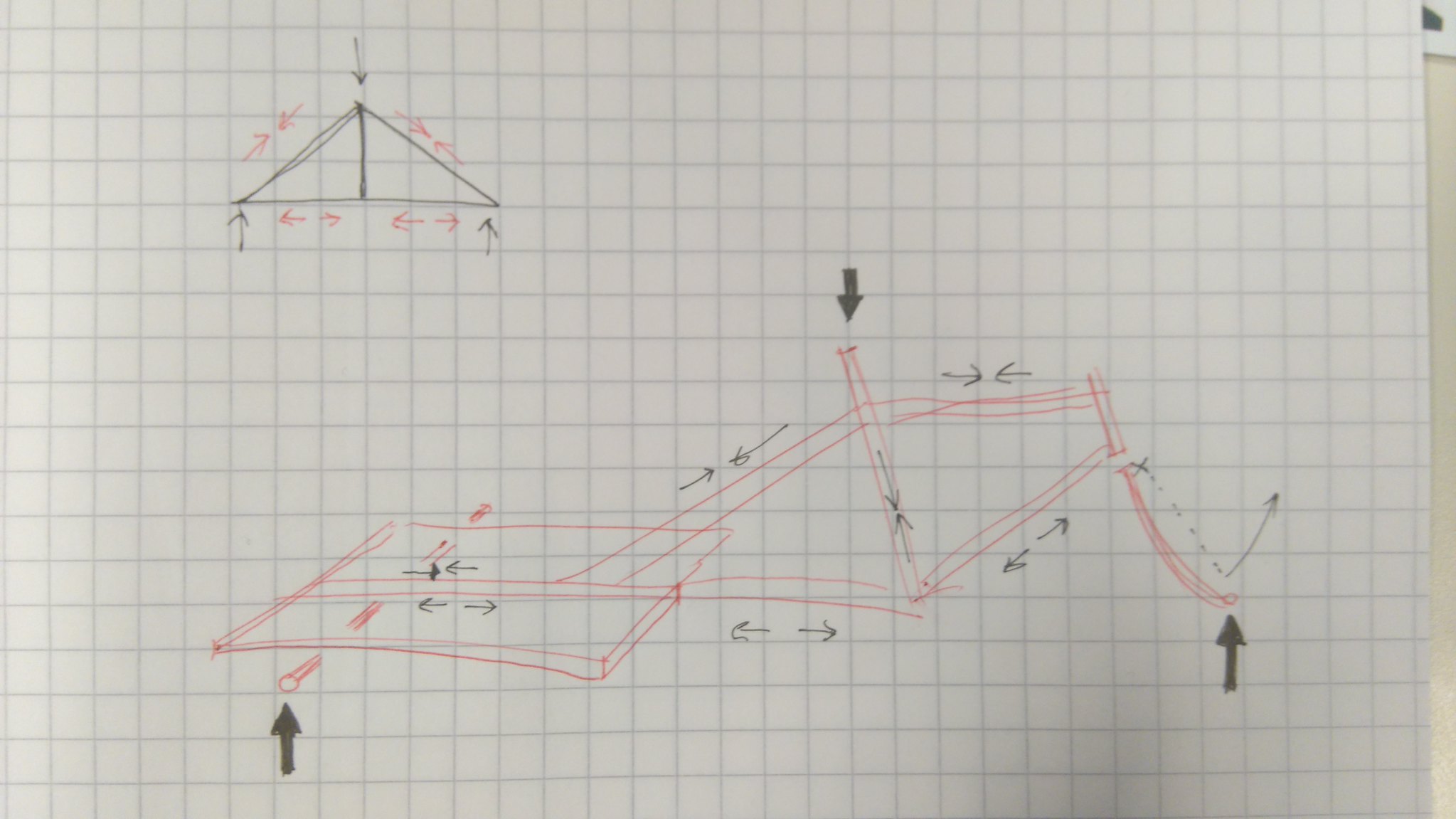This meticulously detailed drawing is sketched on graph paper, identifiable by its small white squares intersected by gray lines. In the upper left corner, a bisected triangle features a vertical line running through its center. An arrow at the apex of the triangle points downward. At the triangle's base, two black arrows point upwards from the bottom-left and bottom-right corners. On the left side near the top of the triangle, two red arrows converge towards each other, mirrored by a similar pair on the top-right.

Towards the bottom of the image, there are further directional indications: on the left side, one arrow points to the left and another to the right. On the right side, two red arrows replicate this orientation by pointing left and right respectively.

Below this section lies another detailed drawing. To the left, a shape resembling a rectangular plank features a rod extending horizontally through its left end, capped by a black arrow. Atop this rectangle, two sets of black arrows illustrate opposing forces, with two arrows pointing towards each other and two pointing away from each other.

Adjacent to the right is another rectangular shape, vertically divided by a line. This shape is marked by a downward-pointing arrow at its top and two inward-pointing arrows at the middle. Additionally, a rod extends from the top left of this rectangle, ending in a black arrow pointing upward.